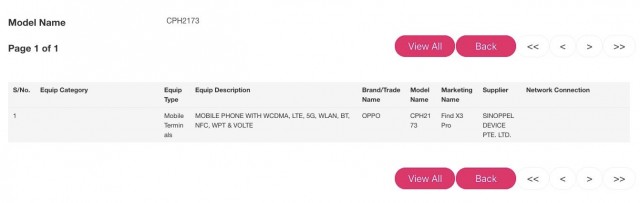A detailed and organized caption for the described image could be:

"The image is a screenshot from a computer interface featuring a document with a predominately white background and black text. It is centered within the frame, providing clear visibility of all text elements. At the top left, 'Model Name' is displayed in bold, accompanied by the number 'CPH-2173'. Directly below, it states 'Page 1 of 1'. 

Within a gray box below, several sections are labeled: 'Equip Category', 'Equip Type', 'Equip Description', 'Brand Trade Name', 'Model Name', 'Marketing Name', 'Supplier', 'Device', and 'Network Connection'. Notable details include 'Mobile Terminals', 'Mobile Phone with Wacoma LTE 5G', 'OPPO', and 'X3 Pro', with supplier information listed as 'Sinopol Device PTE Limited'.

In the top right corner, two reddish-colored oval buttons are positioned: the left one labeled 'View All' and the right one labeled 'Back'. Adjacent to these buttons are sets of navigation arrows: one pair pointing left, one single arrow pointing left, one single arrow pointing right, and another pair pointing right. 

The bottom right corner of the image mirrors this layout, with identical 'View All' and 'Back' buttons, and the same arrangement of navigation arrows, ensuring consistent user interface elements at both the top and bottom of the document."